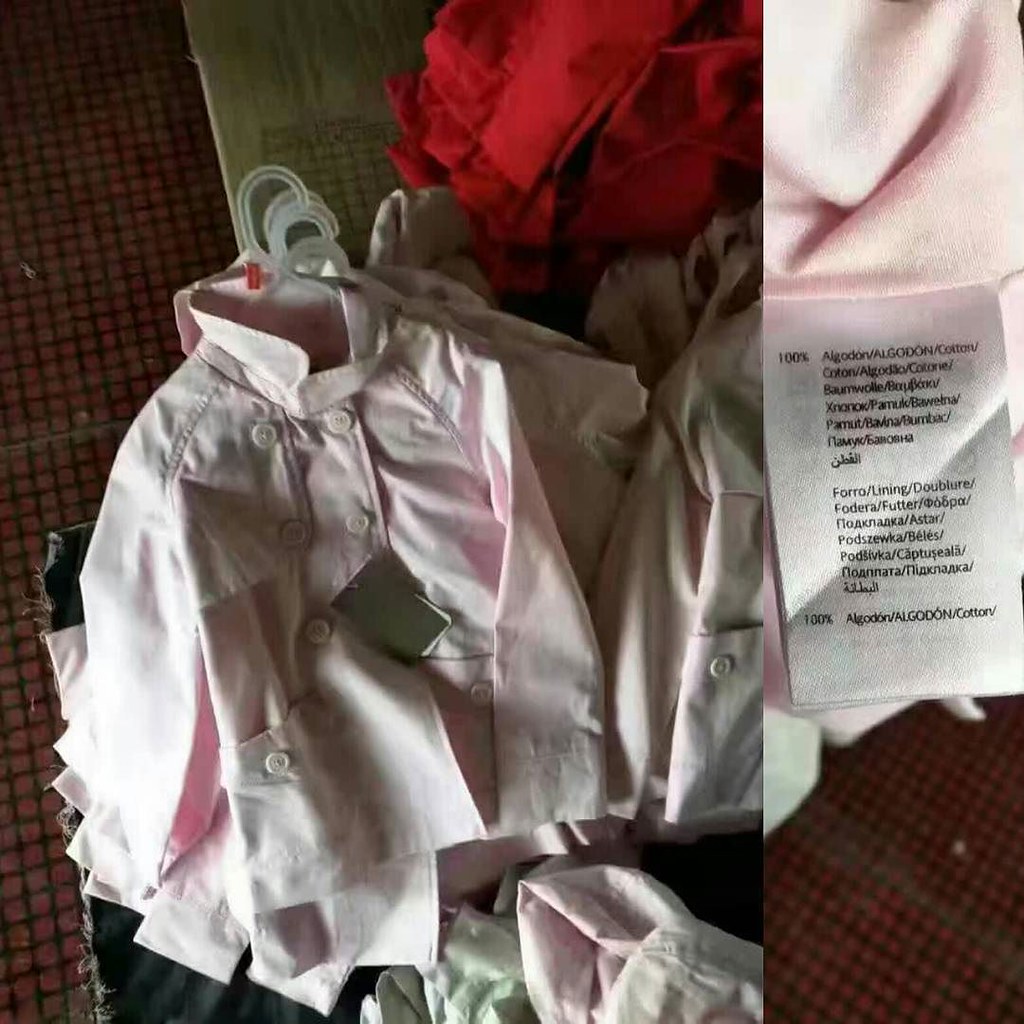This image set consists of two vertically-oriented, rectangular photographs.

The left image showcases a stack of neatly arranged clothing items, all hung on clear plastic hangers. The focal piece at the top of the stack is a light pink jacket adorned with large buttons and accompanied by a black tag. Surrounding this jacket, to the right side, are additional garments in shades of red and white, adding to the layered texture of the display. The floor beneath the stack presents a striking red and black checkered pattern, which contrasts sharply with the pastel tone of the jacket and adds a vintage touch to the scene.

The right image is a narrower, close-up shot focusing on the black tag of the light pink jacket. The tag itself contains text written in a foreign language, though the specific language is not identified in the details. This close-up provides a glimpse into the brand or specific details of the jacket, adding an element of intrigue and highlighting the craftsmanship of the piece.